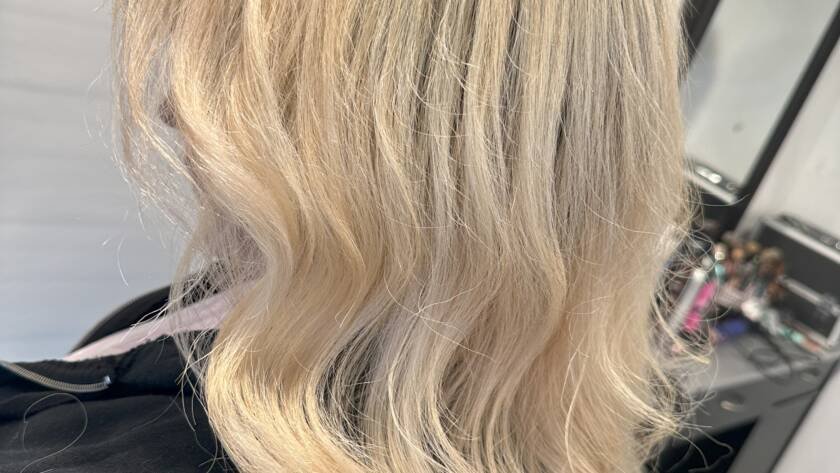In this full-color photograph taken indoors with artificial lighting, we observe an intimate scene inside a hair salon. The horizontally rectangular image predominantly features a blonde-haired woman in profile, though her face is mostly obscured by her flowing, corn silk-colored hair, which has a subtle wave and a slight fuzziness, with wisps trailing down. Her complexion hints at being Caucasian, and you can just make out the tip of her nose and lips. She is dressed in a black top, which could be a sweater or hoodie. 

The background on the left side of the image is a plain white wall, contributing to a clean and uncluttered space. In contrast, the right side of the frame is occupied by a gray countertop that holds various hairstylist supplies, including some bottles and black cords, partially captured in the reflection of a black-framed mirror above the counter. The items on the counter are slightly out of focus, emphasizing the central figure's hair and the serene atmosphere of the salon setting.